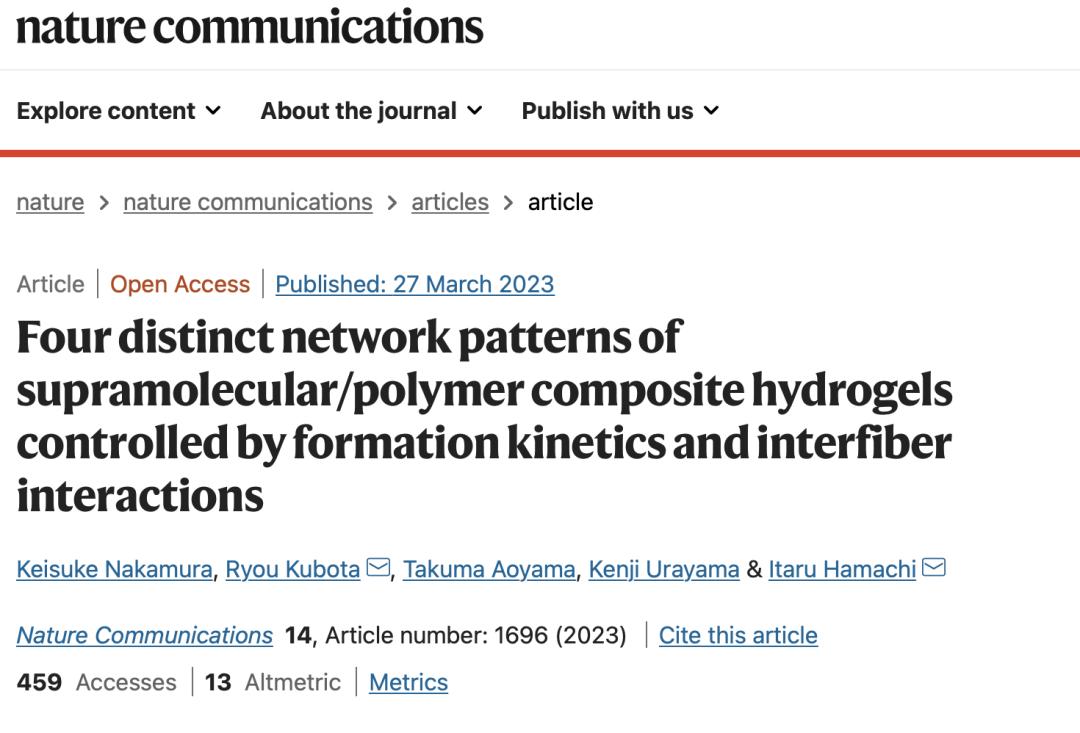This is a detailed caption providing a thorough description of the webpage layout for an article found in the Nature Communications Journal:

---

At the top of the webpage, there is a navigation bar in black lettering featuring options such as "Explore content," "About the journal," and "Publish with us," each accompanied by a drop-down arrow for additional options. Just below this, a red line demarcates the navigation area from the rest of the page.

Beneath the red line, the headings "Nature," "Nature Communications," and "articles" are displayed, with "article" in bold. Proceeding down, the page indicates the article's type as "Article" and specifies "Open Access" in orange text. The publication date, "27 March 2023," is shown in blue, suggesting it is a clickable link.

The headline below these details reads, "Four distinct network patterns of supermolecular polymer composite hydrogels controlled by formation kinetics and inter-fiber interactions." This is followed by the list of five authors, whose names are in blue and also serve as links. Beside two of the authors' names, there is an envelope icon, allowing for direct contact via email.

At the very bottom, "Nature Communications" is again shown in blue, indicating a link, along with an article number and a citation link for referencing the article.

---

This caption encapsulates the layout and visual hierarchy of the webpage, highlighting clickable elements and key features for easy navigation.